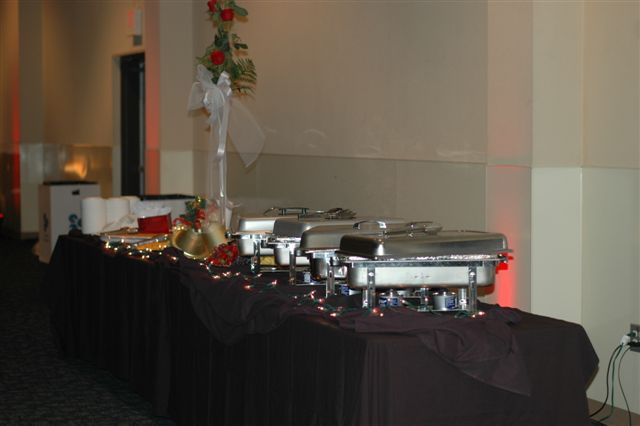This color photograph captures an indoor event, likely a holiday luncheon at a hotel or similar venue. The room features white and gray, off-white colored walls adorned with festive decorations, including a Christmas ornament with red bulbs, green leaves, and a large white bow. A long table, or perhaps two joined together, dominates the scene, draped in a dark blue (or black) tablecloth that nearly reaches the floor. This table serves as a buffet, with several silver heating trays accompanied by Bunsen burners to keep the food warm. Near the bottom of the setup, colored Christmas lights add a festive touch. 

On the left side of the image, you can spot an exit door with a sign above it and an adjacent trash or recycle can. There are plates, cups, and bowls neatly stacked, ready for guests. Additionally, an electrical outlet with three cords plugged in can be seen on the right side, suggesting some equipment requires power. The overall decor and arrangement give off a warm, celebratory atmosphere consistent with a self-serve buffet setting.